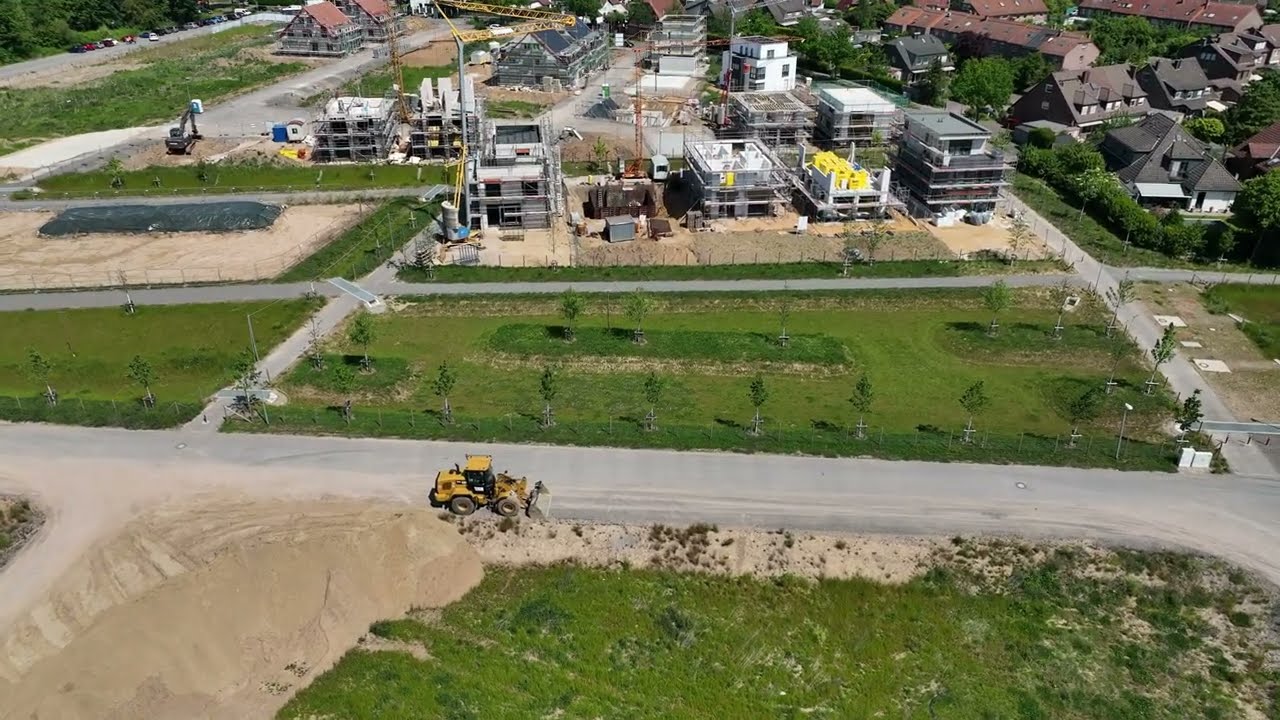The image captures a suburban construction area from a high perspective, likely taken by a drone. In the foreground, there is a grassy field with a sandy patch on the left edge, intersected by a small path leading off from a road. To the right of this grassy field is a yellow construction vehicle, possibly a tractor, situated along a curved road. Beyond this area, another grassy field is lined with trees and bordered by paved roads.

Further into the image, a large construction site is visible, featuring several buildings in various stages of completion, with some structures reaching upwards of five to six stories. Cranes are positioned among the half-built buildings, which are clustered together. This construction site is flanked by additional plots of land, some still sandy and undeveloped, while others show signs of ongoing construction.

On the right side of the image, a residential neighborhood with large houses and abundant trees appears. Multiple small roads connect these different sections, creating a network of pathways linking the suburban landscape. In the distance, more construction activity is visible, indicating further development in the left-hand side of the image.